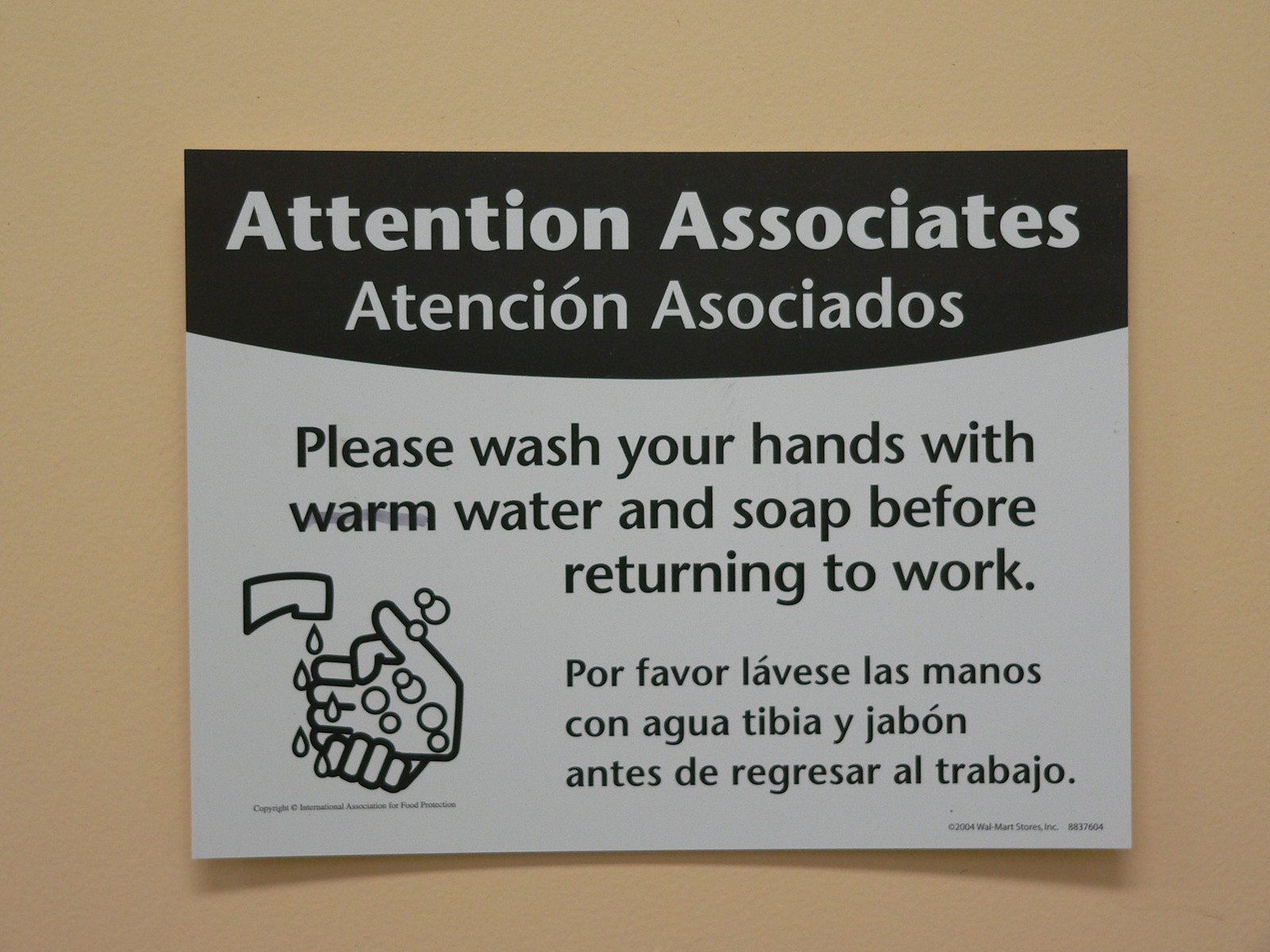The image showcases a sign mounted on a pale beige or white wall, with a rectangular design divided into distinct sections. At the top, set against a black background, bold white letters announce, "Attention Associates," followed by the Spanish translation, "Atención Asociados." Beneath this header, on a white background, is a crucial hygiene reminder: "Please wash your hands with warm water and soap before returning to work," again reiterated in Spanish as, "Por favor, lávese las manos con agua tibia y jabón antes de regresar al trabajo."

A simple yet informative graphic is included, depicting hands being washed under a faucet, with soap bubbles illustrating proper handwashing technique. This sketch-like drawing is positioned towards the lower left of the sign. Additionally, fine print is discernible in the bottom corners, though too small to read clearly. Notably, someone has faintly marked a line through the word "warm" in the English instruction, drawing subtle attention to this detail.